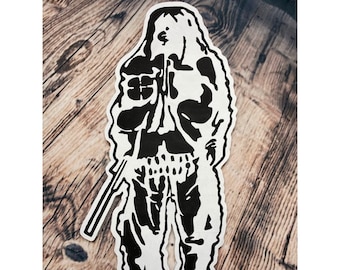The image is of a black and white sticker set against a diagonally-patterned wood background with a high-contrast wood grain. The wood appears antique and distressed, featuring visible knots and gradients. The sticker itself depicts a silhouette of a man with long hair and a beard, possibly holding a shotgun or rod in one hand. The figure is intricately detailed with abstract shapes over the body, including what resembles a skull on the torso, and is wearing a jacket and very baggy pants. The silhouette has a white outline with black splotches that accentuate certain areas, giving it a dynamic, almost shadowed appearance. It seems to be a paper cut-out placed over the textured wooden background.